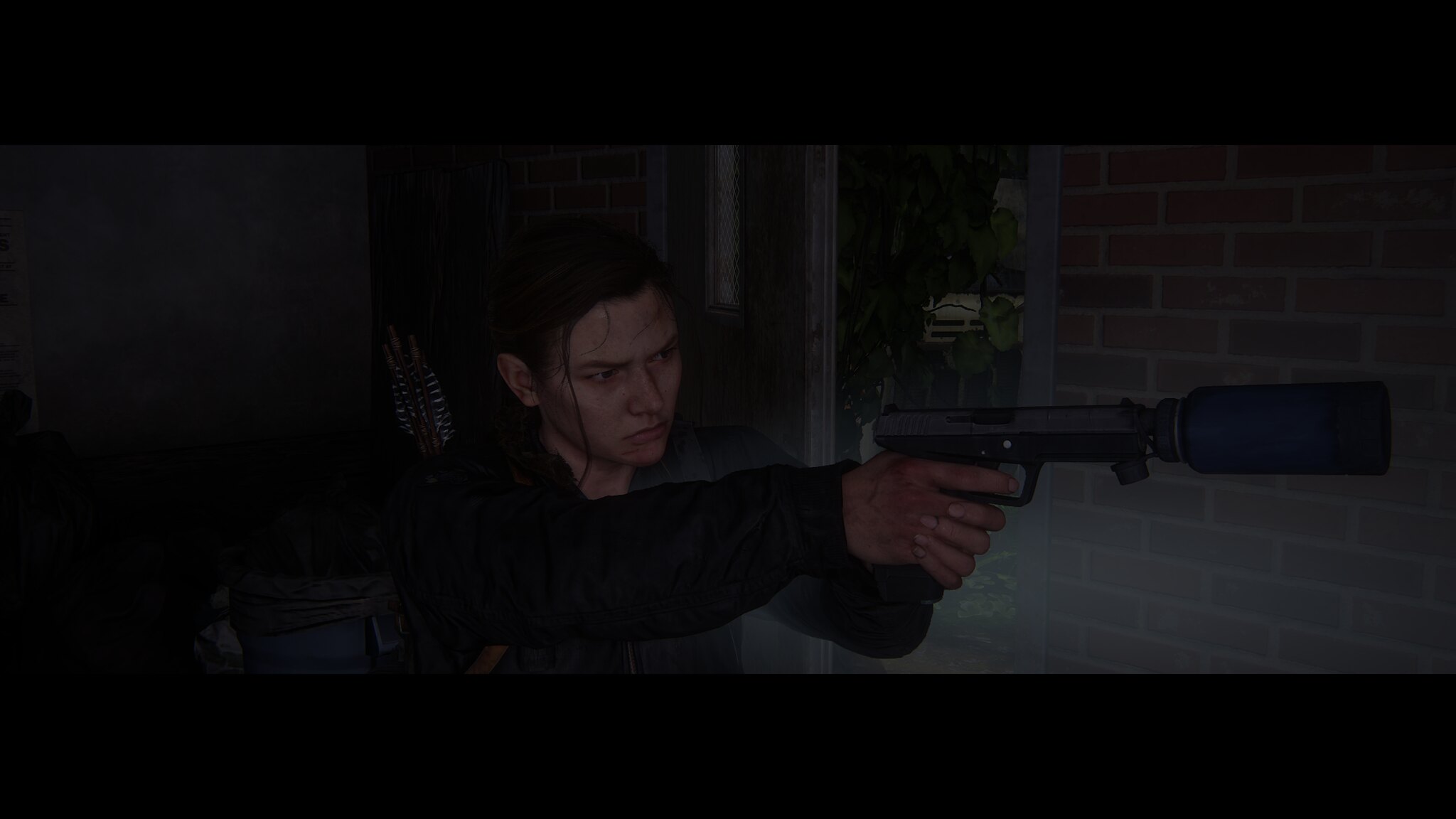In this dark, moody photograph, a person with long hair stands outside a red brick house, which has black strips along its top and bottom edges. The house features a window with a white sill and a touch of whitish color at the base. The person, wearing a long-sleeved black shirt, holds a large gray and black gun with an attached cylindrical silencer, aiming it seriously ahead. In the background, a trash can and a white garage door are faintly visible, adding to the scene's tension and somber atmosphere.